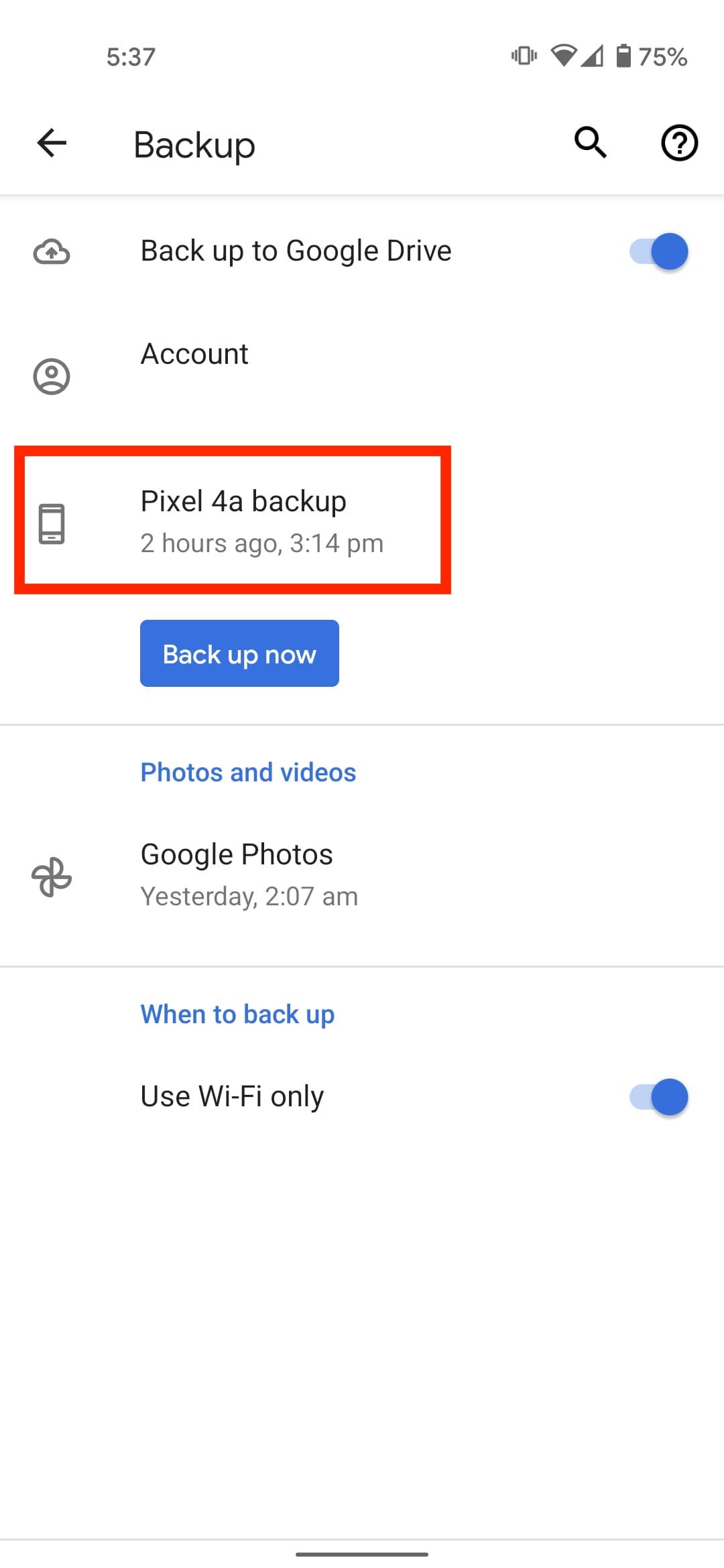In this image, what appears to be a screenshot of an Android smartphone is displayed. The top of the screen shows the current time, 5:37, along with indicators for Wi-Fi connectivity, signal strength, and battery level at 75%. The screen is titled "Backup" and features a magnifying glass icon and a circled question mark icon in the top corners.

Moving down, there is a section labeled "Backup to Google Drive," which is turned on. Directly below, the section "Account" is visible, followed by "Pixel 4a backup," with a smaller line of text beneath that reading "2 hours ago, 3:14 PM," enclosed in a red box. A blue button labeled "Backup now" in white text is placed below this section.

Further down, in blue font, the words "Photos and Videos" are displayed, followed by "Google Photos" in black font with a timestamp of "Yesterday at 2:07 AM." Below this, another blue-font line, "When to backup," is shown. The final line in black font reads "Use Wi-Fi only," which indicates that this option is turned on.